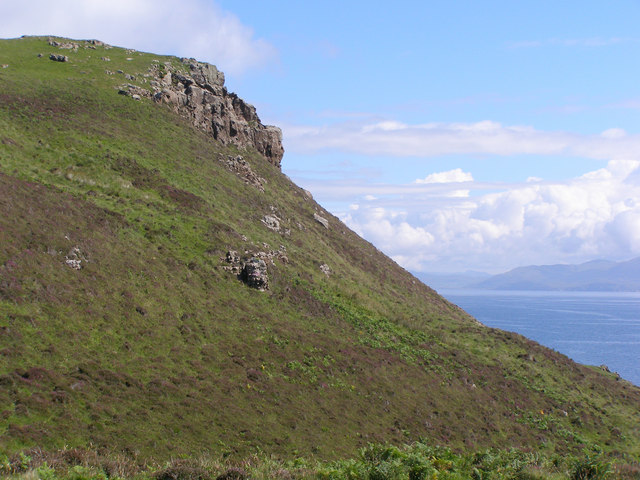This image is a color photograph captured from a drone, offering a slight downward view of a rugged outdoor landscape. The foreground is dominated by a craggy, grass-covered hillside that slopes from the upper left to the lower right corner of the image. The hill is sparsely vegetated with patches of green grass, some brown dirt, and scattered rocks. A jagged rocky ledge is prominently visible near the crest on the left, while the rest of the hillside smooths out as it descends. On the right-hand side of the photograph, a vast body of smooth blue water, possibly an ocean, bay, or large inlet, stretches across the background. In the hazy distance at the horizon line, another landmass resembling the craggy hill in the foreground can be seen, shrouded in mist with indistinct details. The sky above is a vibrant blue, dotted with white puffy clouds, contributing to the overall sense of immense scale and natural beauty. A small bird, possibly a seagull, is captured in flight at the top right, adding a dynamic element to the serene and picturesque scene.